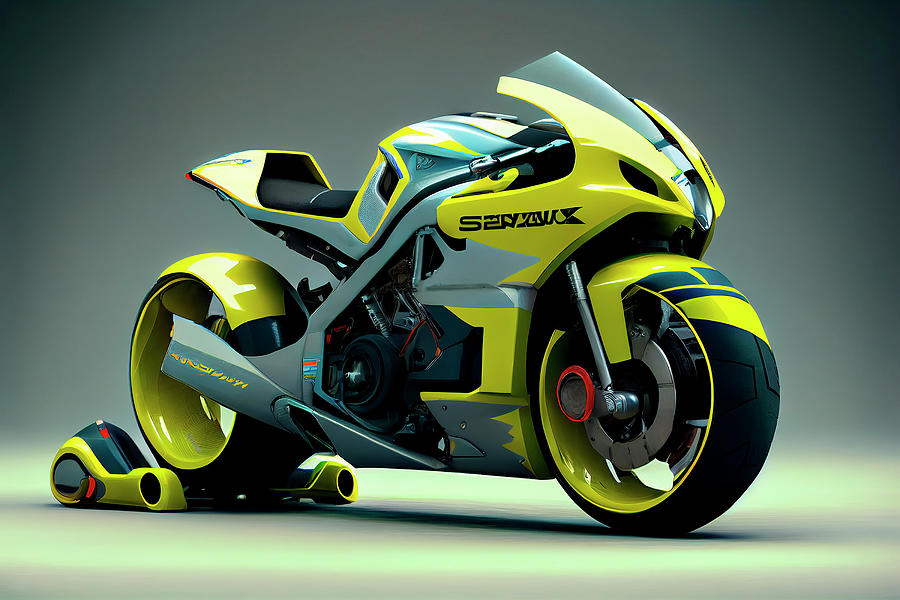The rectangular image, broader than it is tall, features a striking blend of green hues as the backdrop, ranging from deep forest green to a light pastel yellow-green. Dominating the center is an eye-catching motorcycle-like bike, which could either be a genuine vehicle or a highly detailed digital rendering. The bike, modern and sleek in design, stands out with its vivid yellow color accented by pastel green highlights. Though partially obscured, the letters "S2" are visible on the bike, hinting at its model or brand. The bike rests on an unusual device attached to its back leg, likely a charger, suggesting it may be an electric bike. The front wheel resembles that of a standard motorcycle, featuring a black and yellow color scheme, while the rear wheel boasts a sophisticated, high-tech appearance, enhancing the bike's futuristic allure.